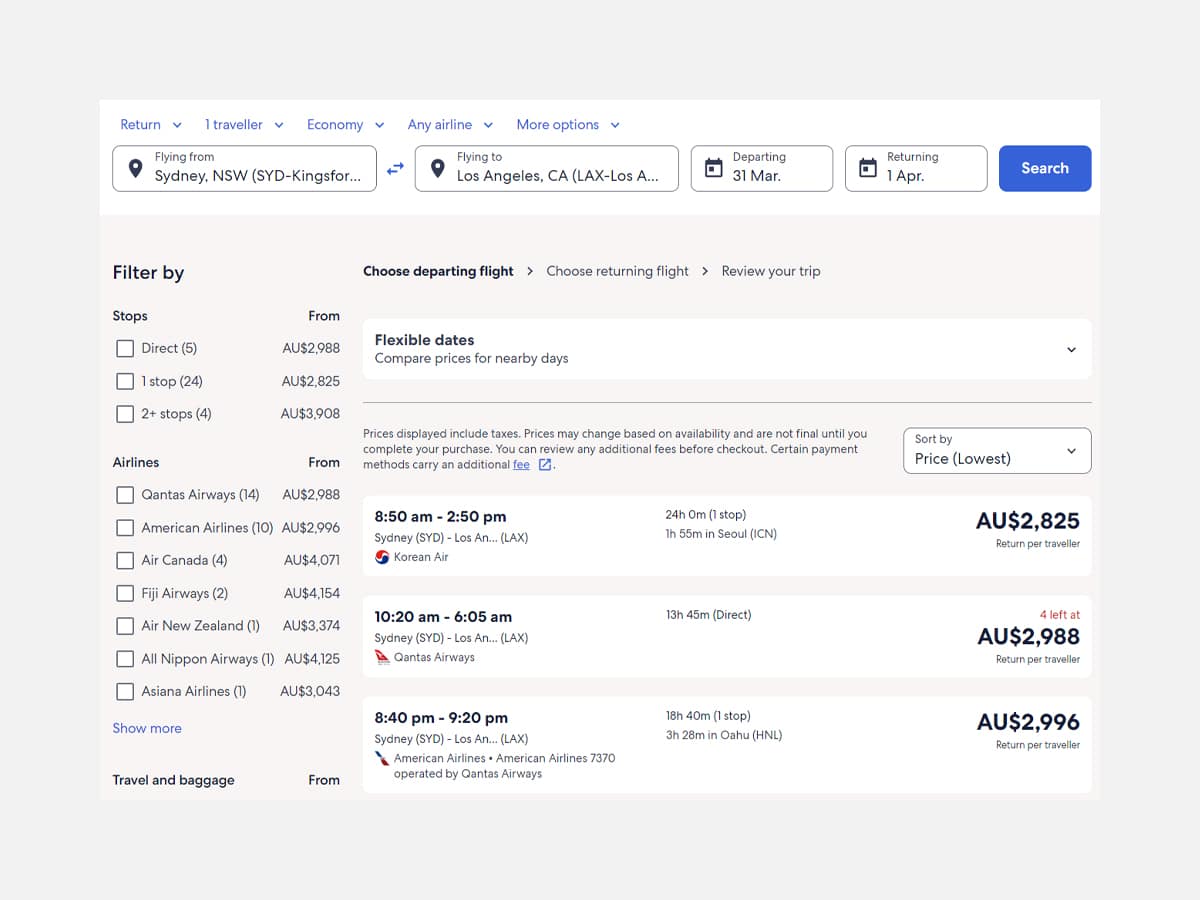The image depicts a section of a travel website designed for booking flights. The website has a clean, white background with predominantly black text and some blue text for specific selections. 

At the top left corner, there's an indication that the user is a return traveler and the options include "Economy," "Any airline," and additional exposures or options. There are five blue tabs near the top of the page, each representing different selectable categories.

Below the tabs, there are fields for flight details. The departure city is listed as "Sydney, NSW (SYD - Kingsford)," although the "D" in "SYD" is cut off. The arrival city is "Los Angeles, California (LAX - Los Angeles)," with "Angeles" partially cut off. 

Next to the city fields, there's a "Departing" date set to "31 March" and a "Returning" date set to "1 April." A blue search button with white text is available to initiate the search.

On the left side, there are filtering options labeled "Filter by," which allow users to refine their search by the number of stops, specific airlines, and baggage options.

To the right, there's a multi-step booking process listed as "Choose departing flight," "Choose returning flight," and "Review your trip." A drop-down box labeled "Flexible dates" is also present.

At the bottom, three different flight options from Sydney to Los Angeles are displayed.